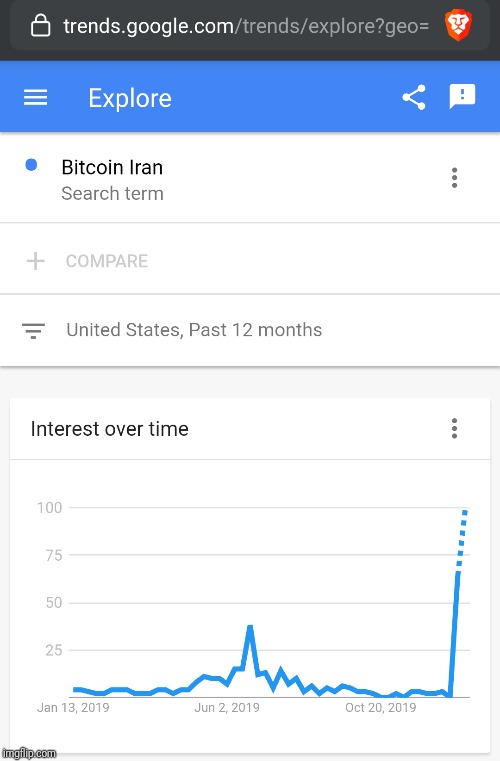The image displays a line graph detailing the search interest for the term "Bitcoin Iran" over time. The URL of the webpage, trends.google.com/trends/explorer, is visible at the top, indicating the source of the data, and a small Brave browser logo is situated in the top right corner. Beneath the URL, a blue navigation bar features the word "Explore" in white text, an options button represented by three horizontal white lines on the left, and share and report buttons on the right.

The graph specifically illustrates the search interest for "Bitcoin Iran" over the past 12 months within the United States. The line representing this data is colored blue. The x-axis of the graph spans from January 13, 2019, to October 20, while the y-axis represents the level of search interest, with a notable spike occurring near the end of the period, around October. The image itself is vertically oriented, further emphasizing the upward trend in search interest seen towards the graph's conclusion.